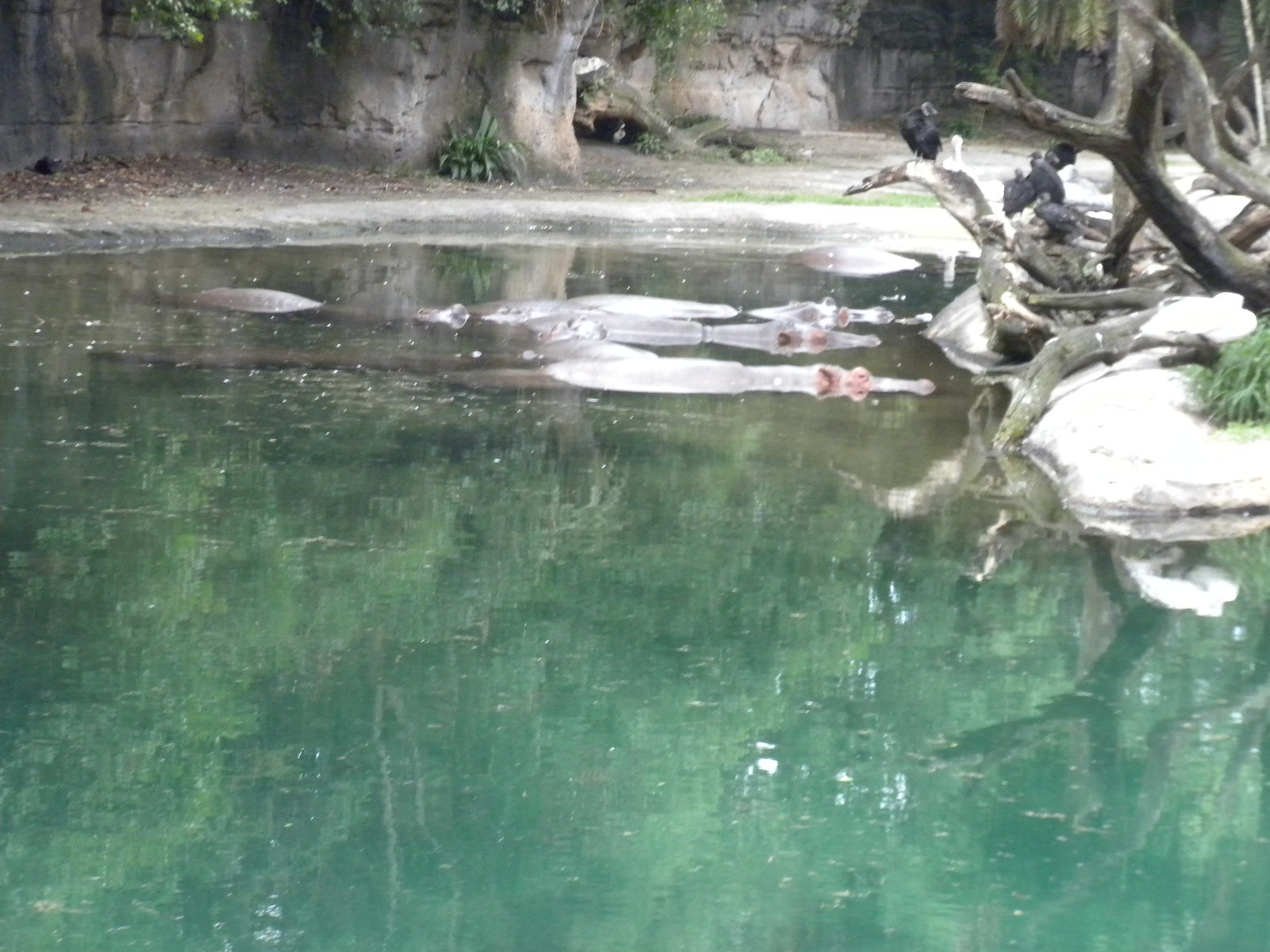The image captures an artificial zoo enclosure designed to resemble a natural habitat, featuring a calm, jade-colored lagoon that dominates the scene. The water, reflecting nearby tree trunks and treetops, appears serene with a blue-green hue. The back wall is molded concrete that mimics nature, complemented by patches of green vegetation and hanging vines. On the right side, large rocks and petrified wood branches are strewn across the water, providing perches for several black birds, possibly crows or vultures. In the water, four submerged hippos are visible, with only their eyes, ears, and noses breaking the surface. The overall scene has a desaturated, overcast quality, resembling an older photograph with some parts of the white stone surfaces appearing blown out by the light.